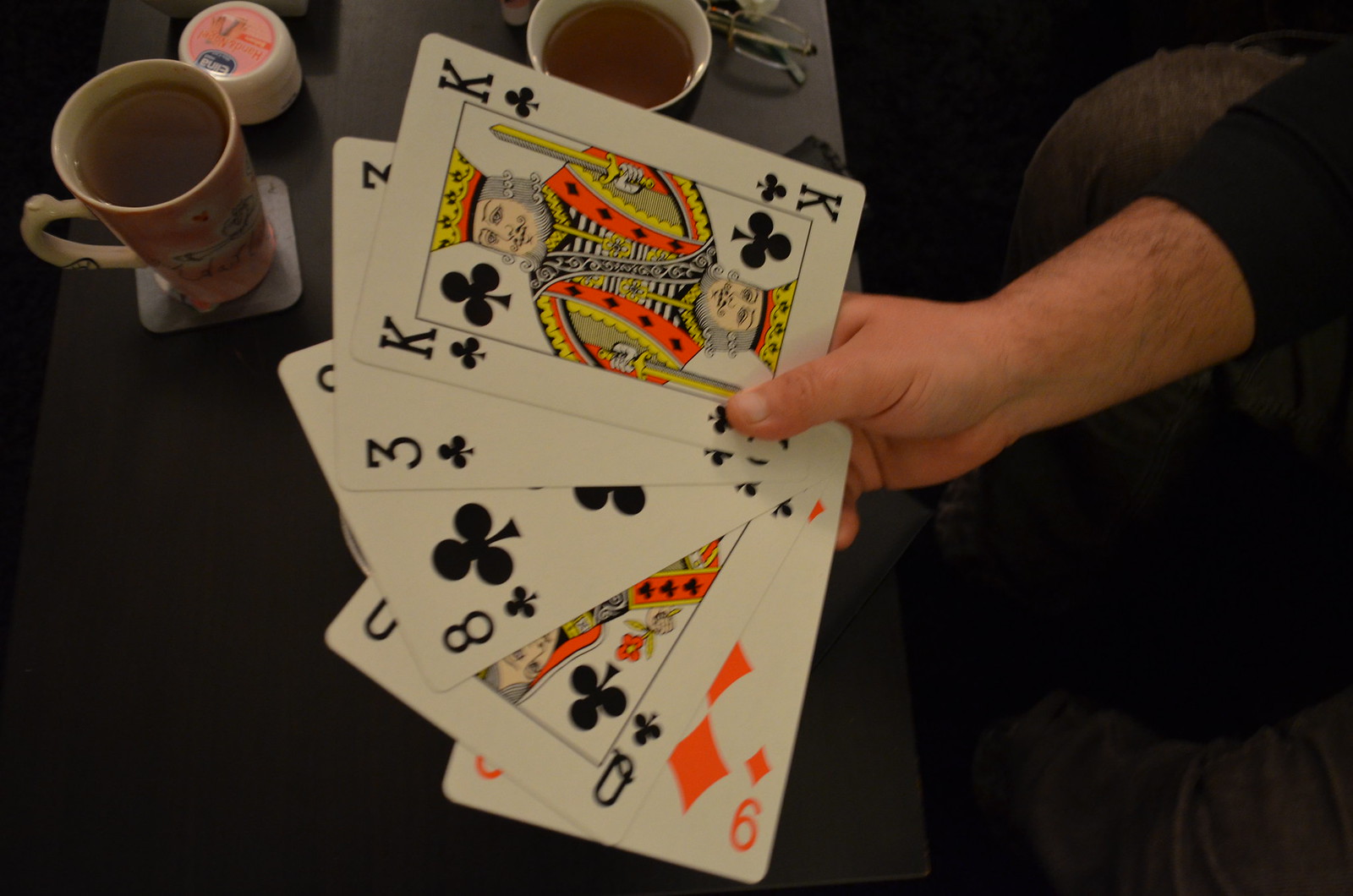In this overhead shot, a person’s hand, emerging from the top right corner of the frame, holds a fan of five large playing cards towards the camera. The hand is clad in a black long-sleeved shirt rolled up to the forearms, paired with dark-colored jeans. The cards on display present a king, three, eight, queen, and a nine of diamonds, with the latter being distinctly red and positioned at the back. Below, a sleek black coffee table is visible, adorned with a few mugs filled with light brown coffee, one of which rests on a rectangular coaster. At the top of the image, a pair of eyeglasses lies on the edge of the coffee table, adding further detail to the scene.